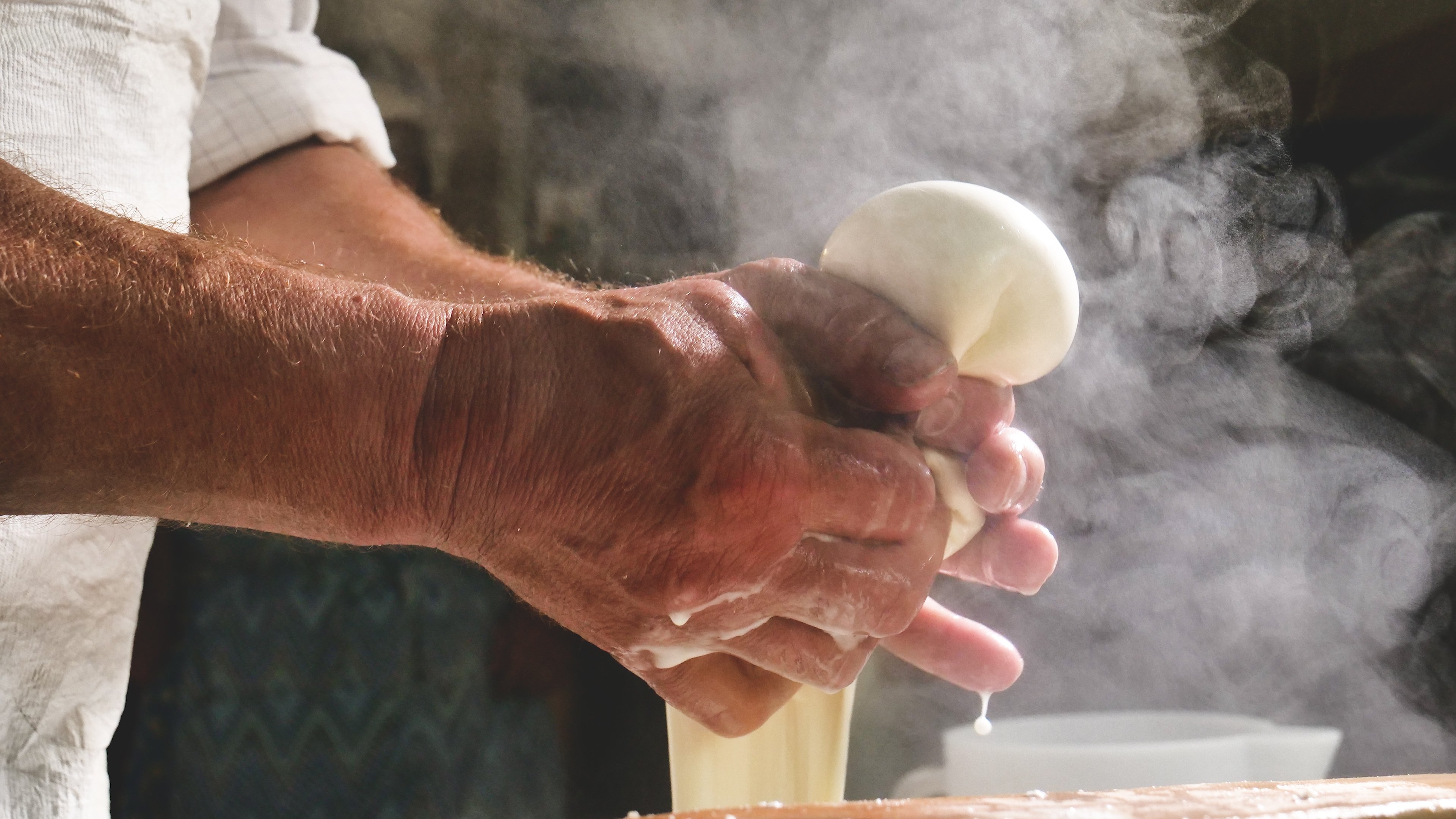In the image, a middle-aged man is in a dimly lit kitchen, focusing on a task that involves both his strong, weathered hands and forearms, which are noticeably hairy. He is dressed in a white shirt with the sleeves rolled up to his elbows. His hands are occupied with kneading what seems to be a soft, sticky dough, which he's lifting and squeezing between his fingers, causing some of the dough to drip in strands and liquid to fall from his hands. Steam or smoke is pervasive in the background, adding a hazy texture to the scene and suggesting heat or fire. The setting includes a green, textured wallpaper behind him, a hint of a tree trunk, and on the wooden table beneath his hands, a half-visible white mixing bowl. The overall atmosphere is one of warmth and rustic activity.